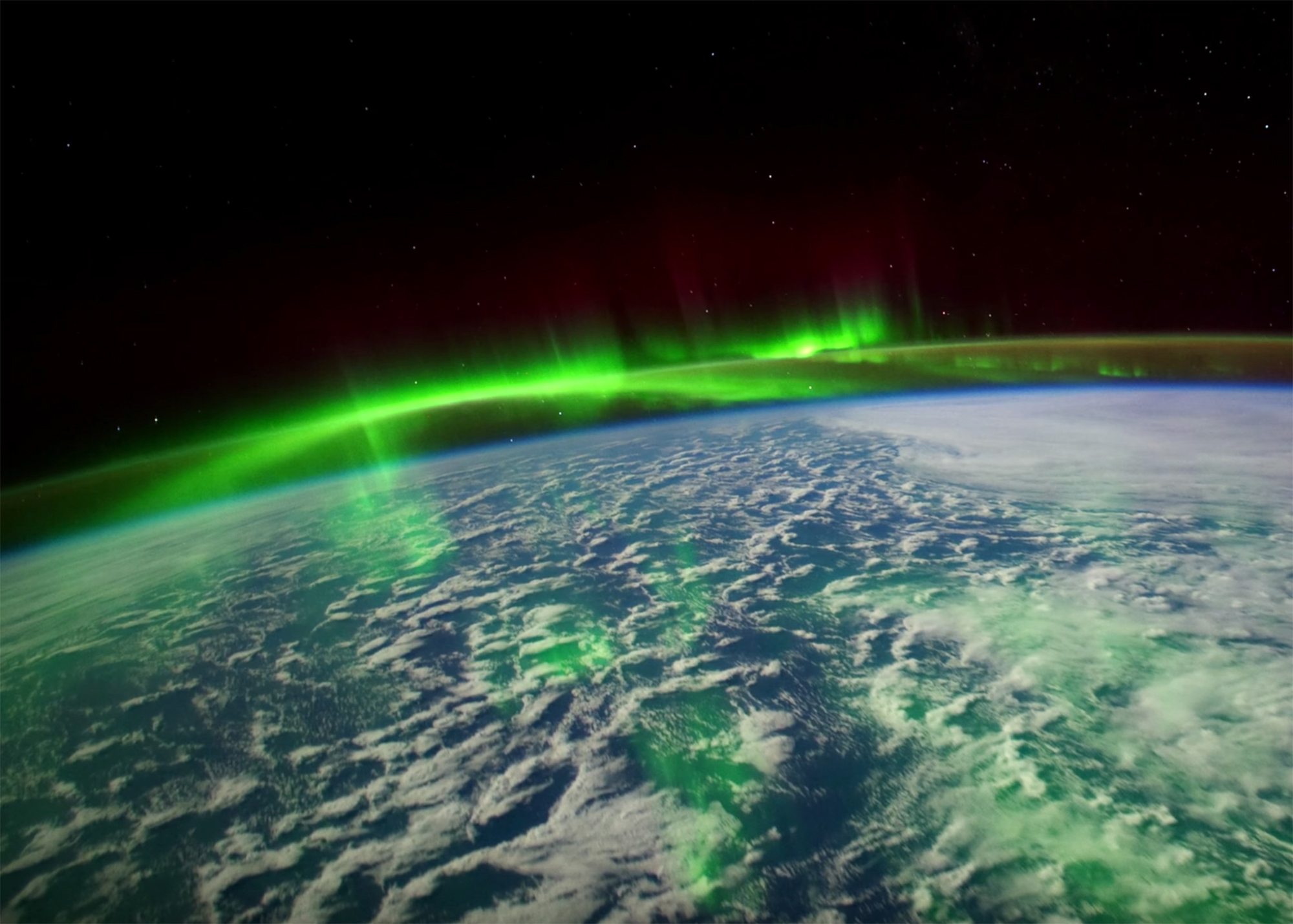This captivating image captures a view of Earth from outer space, showcasing a striking display of what appears to be the Aurora Borealis. The bottom half of the picture features Earth with mostly oceanic blue and white clouds scattered predominantly on the left side, with a larger cloud bank near the upper right. The curvature of the Earth is subtly visible, suggesting a limited section of the globe is shown. Above the Earth, bright neon green lights, reminiscent of the northern lights, fill the atmosphere, extending over the clouds. The top half of the image is a stark black void of space, punctuated by a few distant stars, enhancing the surreal and otherworldly effect of the scene. The juxtaposition of Earth’s tranquil blues and whites with the vibrant green auroras set against the blackness of space makes for a mesmerizing and unique visual experience.